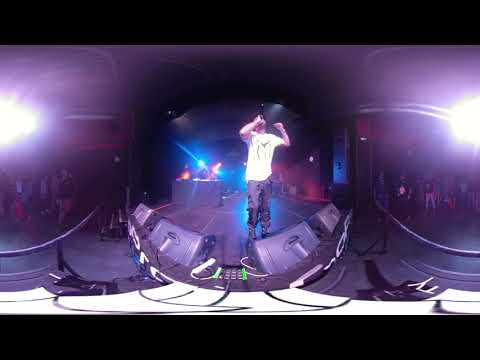The image captures a 360-degree view of a stage performance featuring a central figure—a man wearing black pants and a white short-sleeved shirt, holding a microphone to his face with one hand while the other arm is raised. The venue is predominantly dark, but it is punctuated by bright stage lights, particularly blue, orange, and red spotlights that illuminate the performer. Surrounding the stage are various pieces of equipment, such as amps, speakers, and possibly a booth behind him. On both the left and right edges of the image, there are spotlights that frame the scene, and faintly visible under these lights is a crowd of about 10 to 15 people on each side, watching the performance. In the background, stage fencing and additional equipment contribute to the setting, suggesting a smaller, more intimate venue, possibly for karaoke or a casual concert.